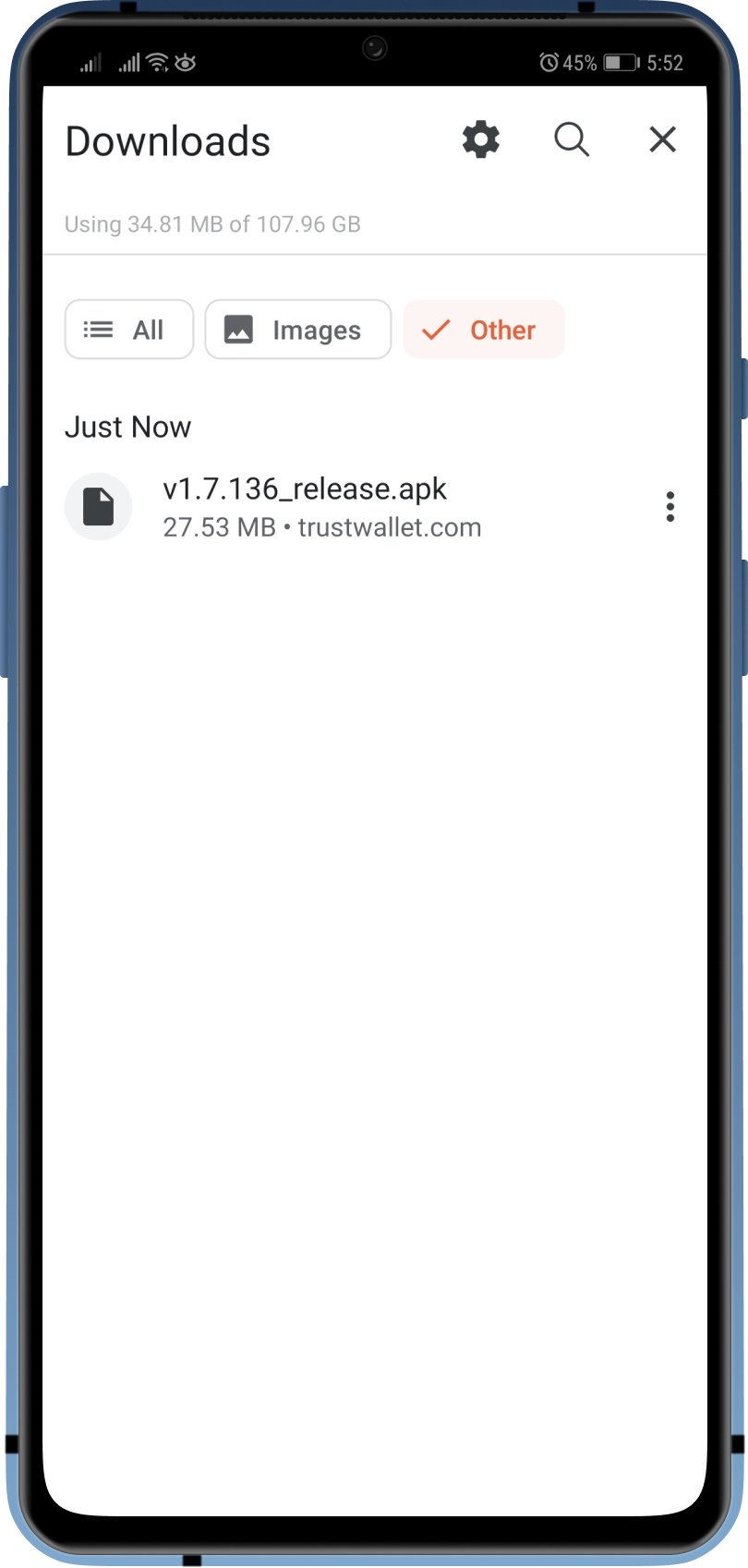The image shows a mobile screen focused on the Downloads section. At the top, a header labeled "Downloads" is accompanied by search and settings icons to its right. Directly below the header, a status bar indicates that 34.81 MB out of 107.96 GB of storage is being used. Three filter tabs—"All," "Images," and "Other"—appear beneath the status bar, with "Other" currently selected. 

The primary display area lists a single download entry: "version 1.7.136-release.apk" from TrustWallet.com, with a file size of 27.53 MB, marked with a timestamp of "just now." 

At the very top of the screen, the phone's status bar shows it is 5:52 PM, with an estimated 45% battery life remaining. Wi-Fi and network connectivity icons are visible in the upper left corner. The overall color scheme is predominantly white with black text.